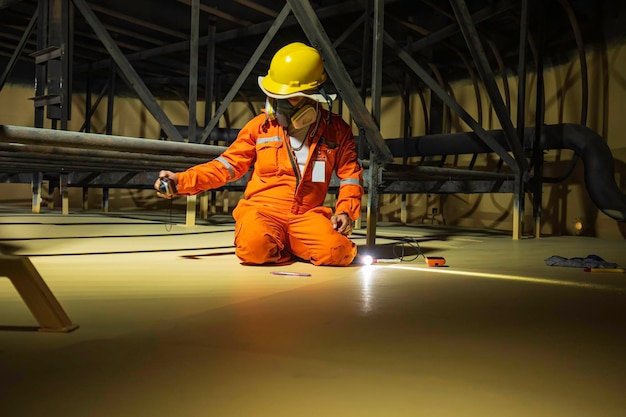The photo, taken from a slightly elevated ground-level perspective, features a construction worker, kneeling on a smooth, shiny beige floor that reflects varying shades depending on the light. The worker, clad in a bright orange jumpsuit with a white shirt underneath and a yellow hard hat, is wearing a white and gray gas mask. They are holding a camera and taking a selfie. The background is filled with dark-colored metal pipes and structures, suggesting an industrial or construction setting. A flashlight lies on the ground to the worker's side, illuminating the scene. Additional items, such as a pin and what appears to be a voltmeter, are scattered nearby, contributing to the cluttered, complex environment of steel frames and piping systems.